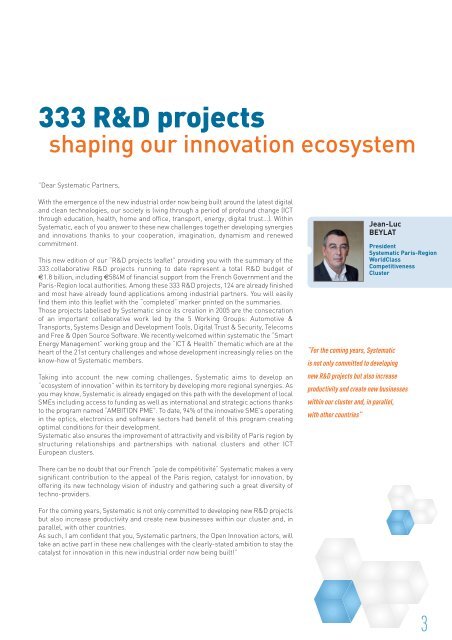The image appears to be a page from an informational mailing, textbook, or magazine. The document is primarily white with text and features the title "333 R&D Projects" in blue font at the top, followed by "Shaping Our Innovation Ecosystem" in orange font just below. At the very top, in small black font, it begins with a salutation, "Dear Systematic Partners," and is followed by five paragraphs of detailed, albeit small, text. On the right side of the page, there is a picture of a middle-aged man in a dark jacket and white button-down shirt identified as Jean-Luc Bailet, President of Systematic Paris Region, with some additional text describing him as a leader in comprehensive world-class research and development clusters. Beneath this is a paragraph in orange text. The bottom section features a series of white and blue cubic or hexagonal blocks, giving a molecular or structural impression, with the number three located in the bottom right corner, presumably indicating a page number.